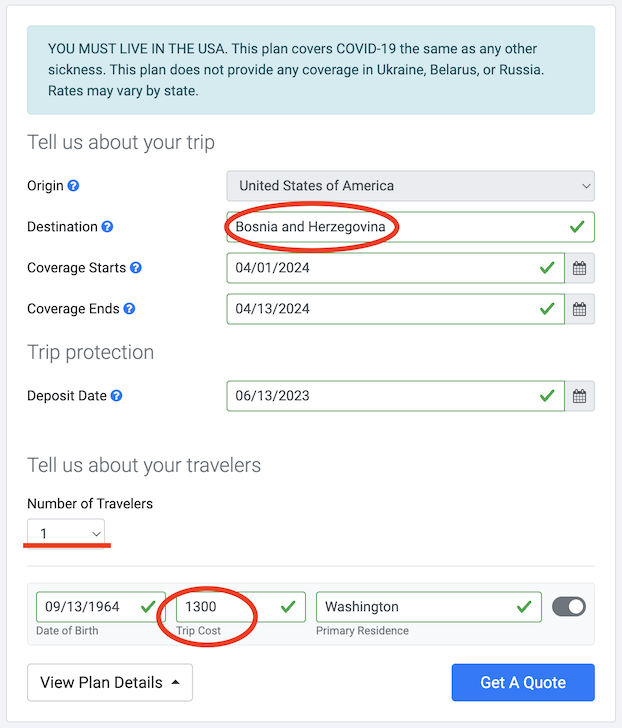**Website Pop-Up: Insurance Plan Details**

**Banner Section:**
- **Appearance:** A prominent blue banner with a lighter shade of blue background.
- **Message (in all capital letters):** "YOU MUST LIVE IN THE USA"
- **Additional Information (regular font):**
  - "This plan covers COVID-19 the same as any other sickness."
  - "This plan does not provide any coverage in Ukraine, Belarus, or Russia."
  - "Rates may vary by state."

**Information Below the Banner (gray font):**

- **Trip Information:**
  - **Origin:** United States of America (selected from a drop-down menu)
  - **Destination:** Bosnia and Herzegovina (selected and confirmed)
  - **Coverage Start Date:** April 1, 2024 (selected from a calendar)
  - **Coverage End Date:** April 13, 2024 (selected from a calendar)
  - **Trip Protection Deposit Date:** June 13, 2023

- **Traveler Information:**
  - **Number of Travelers:** 1
  - **Date of Birth:** September 13, 1964
  
- **Trip Costs:**
  - **Trip Cost:** $1,300
  - **Primary Residence:** Washington (selected and confirmed)
  
- **Action Buttons:**
  - **View Plan Details**
  - **Get a Quote**

This detailed description captures the essence of the pop-up insurance plan section on the website, ensuring clarity and comprehensiveness for users.